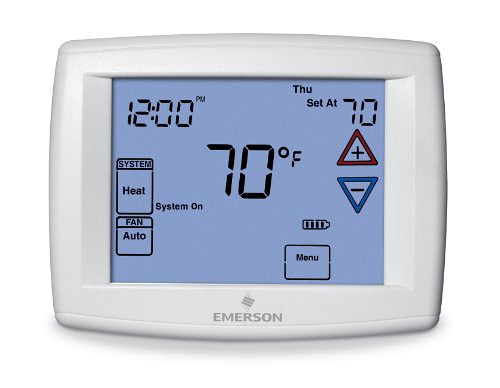The image depicts a close-up view of a rectangular white thermostat. The central feature of the thermostat is a grayish-blue screen with black text and numbers. In the upper left corner of the screen, the time is displayed as "12:00 PM." Below the time display, there are two rectangular sections: the top, longer rectangle reads "system" and "heat," while the shorter rectangle beneath it indicates "fan" and "auto." To the right of these sections, the words "system on" are visible. 

Prominently displayed in the center of the screen is the temperature "70°F." On the right side, "THU" appears in black text, with "set at 70" directly below it. Adjacent to these words are two triangular buttons: one red with a plus sign pointing upwards, and one blue with a minus sign pointing downwards.

Additionally, there is a battery icon, which is a rectangle with a loop on the right side, showing four bars to indicate a full charge. Finally, a square button labeled "MENU" is also present on the screen.